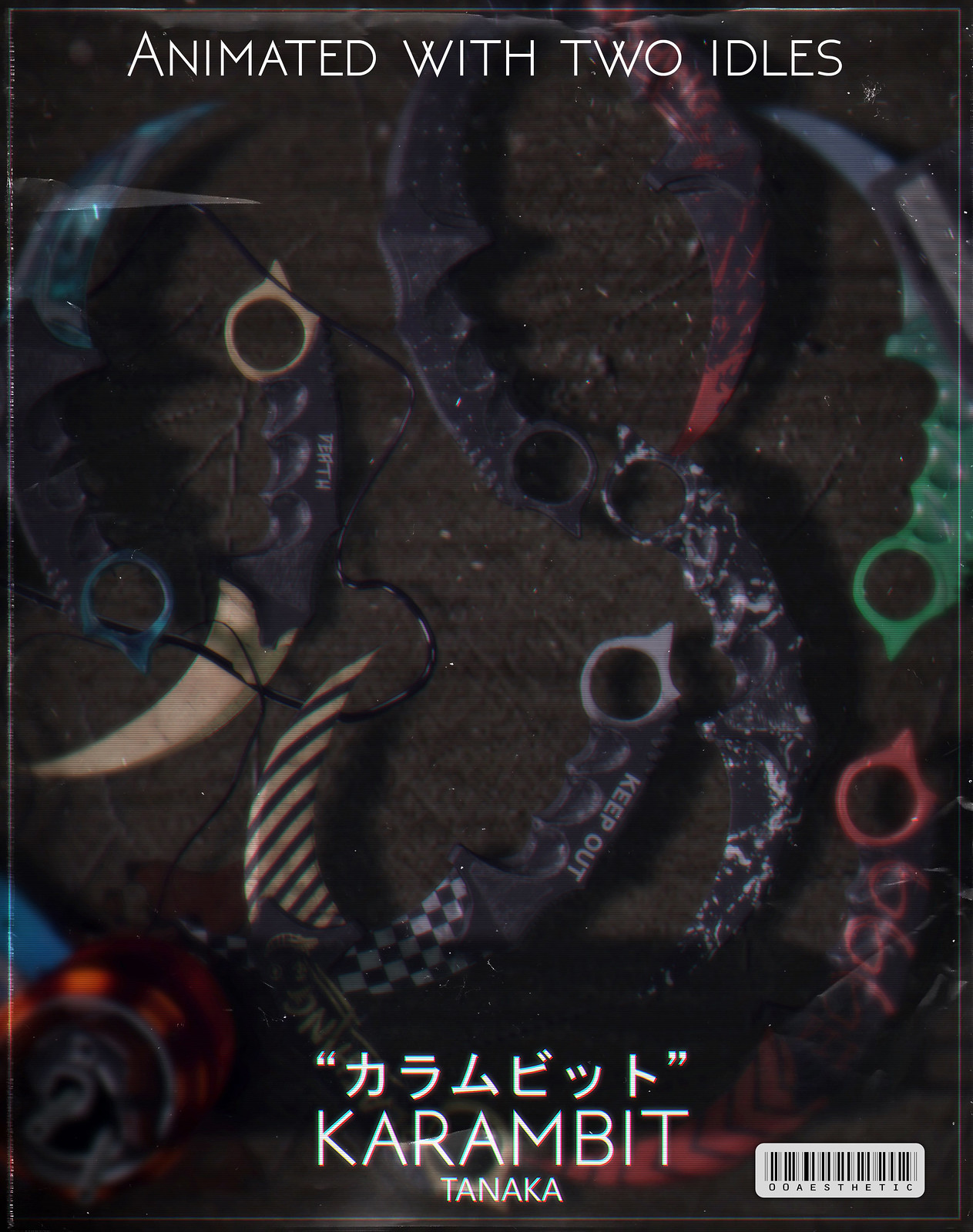The image appears to depict the cover of a book or album. At the top of the cover, there is white text that reads "Animated with Two Idols." Below that, in the middle of the cover, is a prominent arrangement of various karambit knives, each featuring a unique design. The paints used range from light blue, yellow, and green to complex patterns such as black and white checkerboard, camouflage, and black with red speckles. The handles of the karambits have ridges for finger placement and a circular ring at the bottom for gripping. The background looks like a rugged dark green tablecloth or carpet, giving a stark contrast to the colorful knives. Towards the bottom of the cover, there is a text that reads "karambit" and "Tanaka" with some Japanese text in quotations above. Additionally, on the bottom right, there is a barcode with the text "OO Aesthetic."